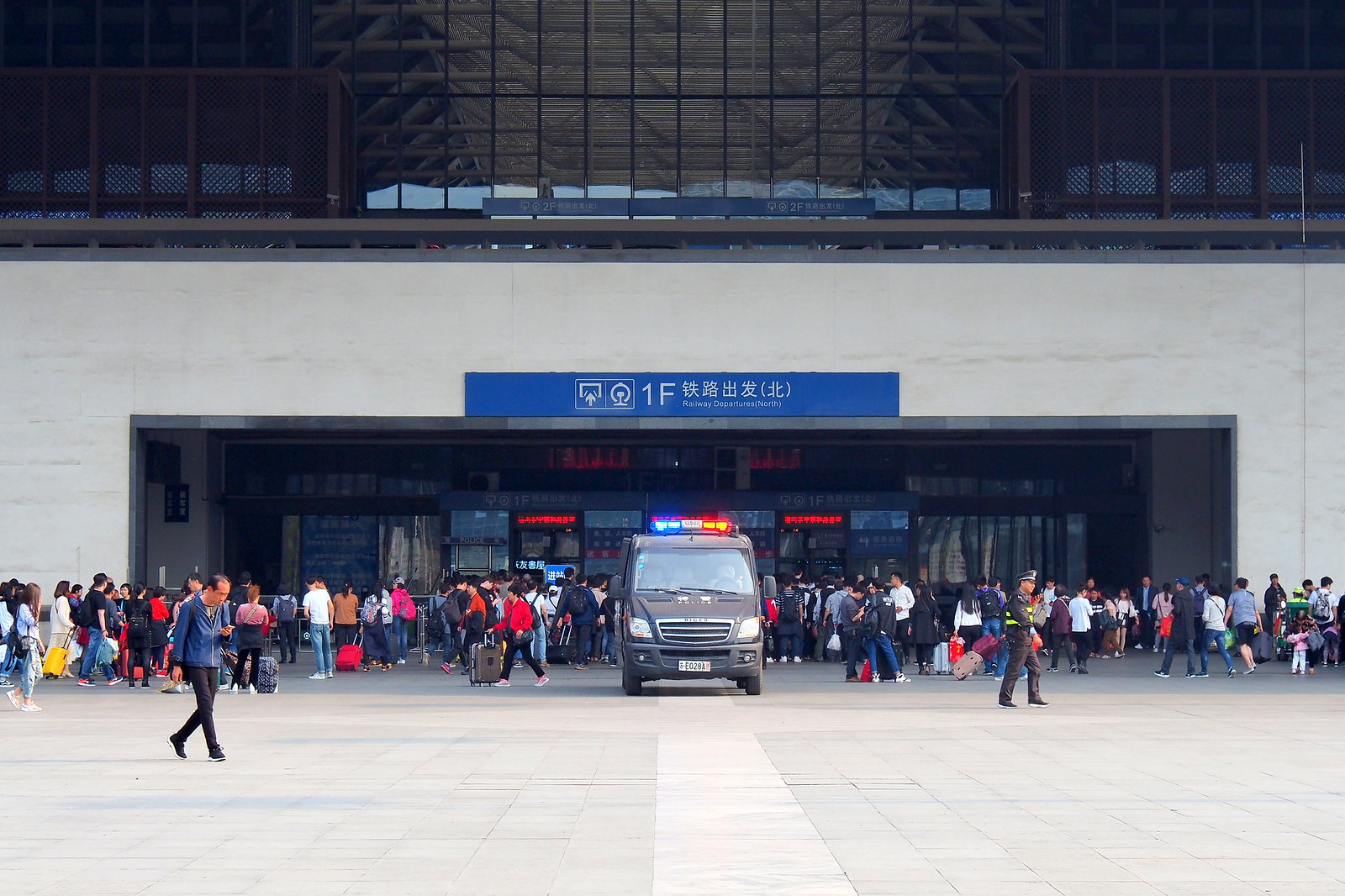The image depicts a bustling scene in front of a large off-white building with a notably wide entrance, reminiscent of an oversized garage door. Prominently positioned in the center is a stationary black police van, distinguishable by its blue and red sirens on the roof and a white rectangular license plate. The entrance is marked by signs, one of which reads "Railway Departure North" in both English and Chinese, suggesting this is a railway station rather than an airport. Surrounding the van is a dense crowd of people, many carrying suitcases and briefcases, indicating a travel-related activity. The lower portion of the image reveals a grey concrete tiled ground, and a police officer is visible on the right side of the van. The scene is animated with approximately a couple hundred individuals casually moving about or standing, filling the frame with a sense of activity and urgency. Large structural beams are visible at the top of the building, adding to the industrial atmosphere of the scene.